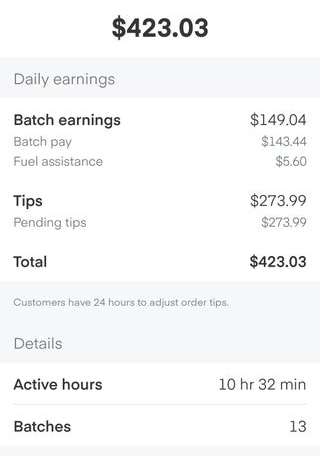The image features a vertical receipt set against a pristine white background. Dominating the top portion of the receipt is a prominently displayed, bold black text showing the total amount of $423.03. Directly beneath this, a gray box provides detailed breakdowns: on the left, it lists "Daily Earnings," followed by "Batch Earnings" of $149.04, split into "Batch Pay" of $143.44 and "Fuel Assistance" of $5.60. Below this segment, the receipt indicates "Tips" of $273.99 with the same figure reiterated under "Pending Tips." 

The "Total," highlighted once again in bold, is shown as $423.03 on the right side of this section. Further down, another grayish box contains an informative note stating, "Customers have 24 hours to adjust order tips." This is followed by a section labeled "Details" which specifies "Active Hours" as 10 hours and 32 minutes and concludes with the number of "Batches" being 13.